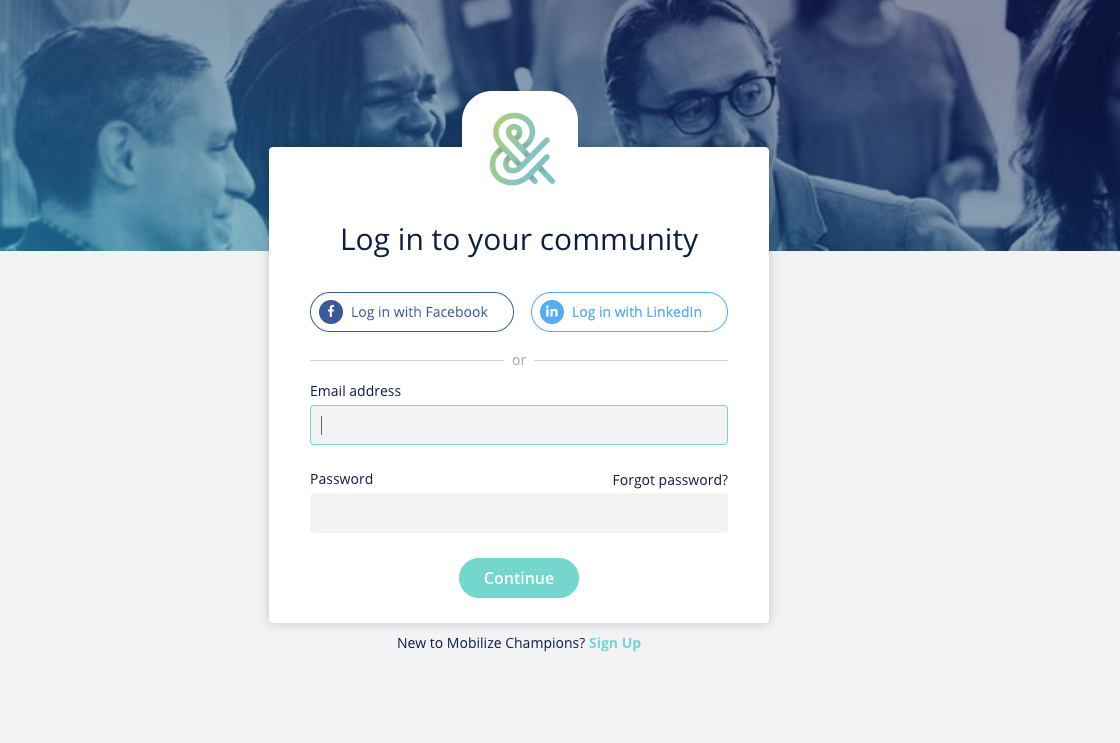The image depicts a login page for a platform named "Mobilize Champions." At the top of the page, there is an illustrative header featuring a crowd of people in blue and gray shades, including a prominent image of a Black man, who appears to have Jewish facial features, suggesting a diverse community. In the background, a smaller image shows a generalized crowd of people.

At the very top of the page, a green '@' symbol is prominently displayed, possibly representing the community aspect of the platform. 

The main section of the page invites users to "Login to your community." Users are given multiple options for logging in: a button to "Login with Facebook," marked with a Facebook icon and a small circle on the left, and another to "Login with LinkedIn," displayed in a lighter blue color.

Below these social login options, there are fields for entering an email address and password, with a "Forgot password?" link positioned neatly at the upper right-hand corner of the password field block.

Finally, a large teal oval button with white lettering says "Continue." Just below this, a message in black lettering reads, "New to Mobilize Champions?" followed by a "Sign up" link in light green, indicating the registration option for new users.

Despite the name "Mobilize Champions" sounding like a video game, the overall design and elements clearly indicate it is not a gaming page but rather a community-focused platform.